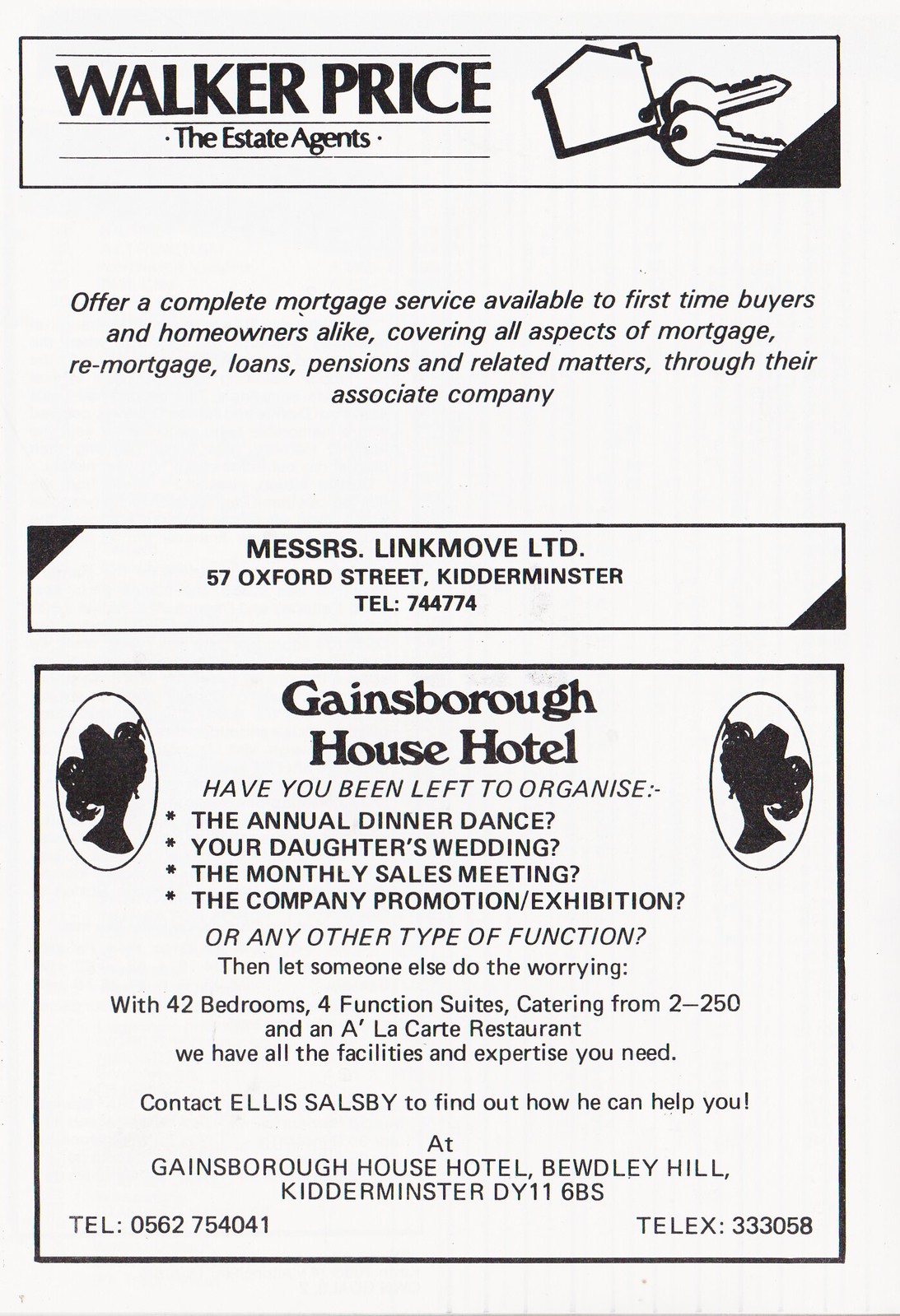The black-and-white advertisement evokes a vintage charm and is meticulously divided into two sections. The upper section prominently features "Walker Price, The Estate Agents" in bold black text within a black rectangle. Accompanying this text is an illustration of a house-shaped keychain with keys, signifying real estate services. Below, in italicized white text, the ad outlines a comprehensive mortgage service for first-time buyers and homeowners, covering various aspects such as mortgage, remortgage, loans, pensions, and related matters through their associated company.

Below this, in another black rectangle, the ad promotes "Messrs Link Movers Limited," located at 57 Oxford Street, Kidderminster, alongside their contact number, 744-774. 

The lower section shifts focus to the Gainsborough House Hotel, framed by a black square featuring text in black. This part of the ad poses a question to the reader about organizing functions such as annual dinner dances, weddings, sales meetings, or company promotions. It highlights the hotel's offerings, including 42 bedrooms, four function suites, catering for 2 to 250 guests, and an a la carte restaurant. The ad encourages contacting Ellis Salisbury for more information, providing the hotel's address at Beadley Hill, Kidderminster, DY 11 6 BS, and contact numbers 0562 75441 and X333 058. Additional elements at the top corners of this section appear to resemble silhouettes, potentially a rooster or a figure's head, giving the layout an intricate vintage touch.